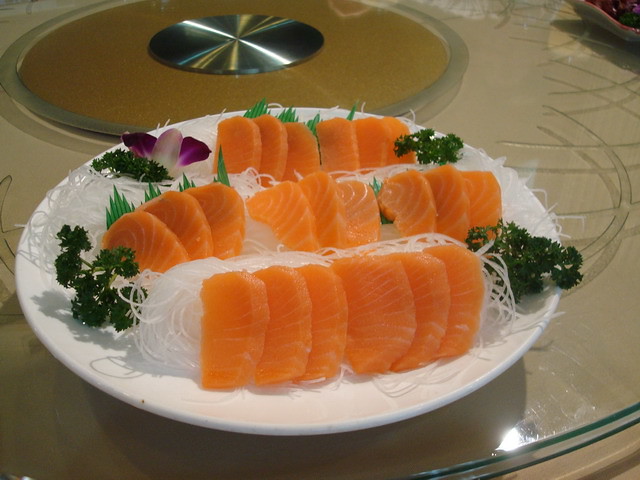The image depicts an artfully arranged plate of salmon sashimi presented on top of a clear, round rotating table, reminiscent of those often found in dim sum restaurants. The creamy white plate features an orderly display of sashimi slices, exhibiting a delicate shade of orange with visible grain lines. These slices are arranged into three rows: the closest row and the farthest row each contain six pieces, while the middle row consists of nine pieces. The sashimi rests on a bed of thin, translucent, whitish rice vermicelli noodles, adding texture and visual interest. Green sprigs, possibly parsley, serve as additional garnish, enhancing the freshness of the presentation. Notably, plastic green grass is subtly placed behind the back and middle rows. To complete the garnish, three delicate flower petals - two purple and one whitish - are artfully positioned in the top left segment of the plate. The entire setup sits on the shiny surface of the rotating table, with the central rotating mechanism visible in the background. The tabletop itself features intricate scrollwork, adding an elegant touch to the overall setting.